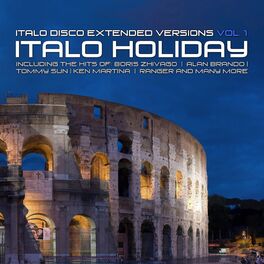The image is a square advertisement for an Italian holiday-themed music compilation titled "Italo Holiday," part of the "Italo Disco Extended Versions Volume 1." The top half of the square is dominated by a dark blue nighttime sky, punctuated by bright blue spots. The top line of text, in small white letters, reads "Italo Disco Extended Versions Volume 1," with "VOL1" also highlighted in blue. Below, the title "Italo Holiday" is prominently displayed in large white letters. The image features a detailed depiction of the Coliseum, stretching from the bottom left corner and extending past the middle of the square. The Coliseum is rendered in light brown and pink hues, with some archways illuminated. Text beneath the title lists the included hits by artists such as Boris Javaru, Alan Durando, Tommy Sun, Ken Martina, Ranger, and many more. In the bottom right-hand corner, a distant scene of buildings on water is visible, adding to the Italian ambiance. The entire composition suggests that this might be the cover for a CD or vinyl record, celebrating Italo Disco music with a vivid Italian backdrop.